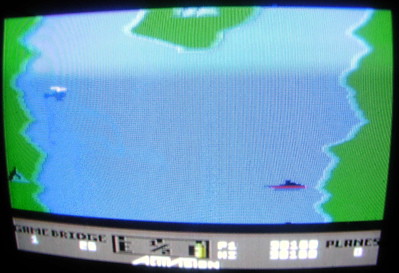The image appears to be a low-resolution screen capture from an early video game. The simplicity of the graphics suggests it could be from the Atari era or an early Nintendo game. Dominating the scene is a blue area likely representing water, flanked by irregular green patches symbolizing land or coastline. In the center of the blue water, on the right, there's a colorful pixelated object with blue and red hues, resembling a ship. Nearby, on the left side, sits a blue and green helicopter with white blades. A solitary pixelated mountain is visible to the left of the water. At the bottom of the screen, a gray strip is labeled "Game Bridge," accompanied by various numbers and the word "planes" with an associated number, further indicating its gaming context.